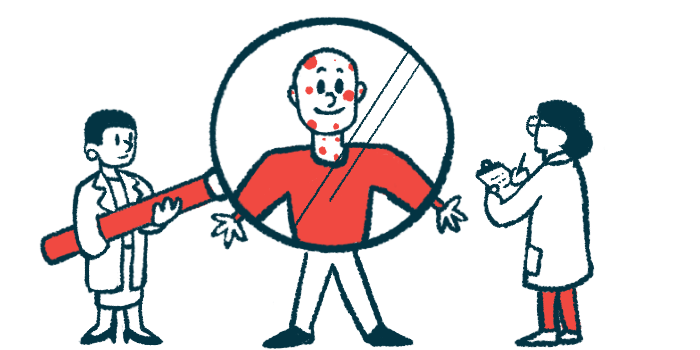The image is an illustration featuring three human figures against a white background, primarily composed of black and white hues, with red accents. In the center, a bald, smiling man with red, measles-type spots on his face and body stands wearing black shoes, white pants, and a red shirt. To his right, a female doctor with black hair and glasses, dressed in red pants, white shoes, and a white lab coat, holds a clipboard and writes detailed notes about the patient's condition. To the man's left, a nurse with short black hair, adorned in white high heel shoes, a white skirt, a white shirt, a white lab jacket, and white earrings, holds a large magnifying glass to closely examine the red spots on the patient. The scene captures a detailed, collaborative medical examination, perhaps aiming to diagnose the man's apparent illness.